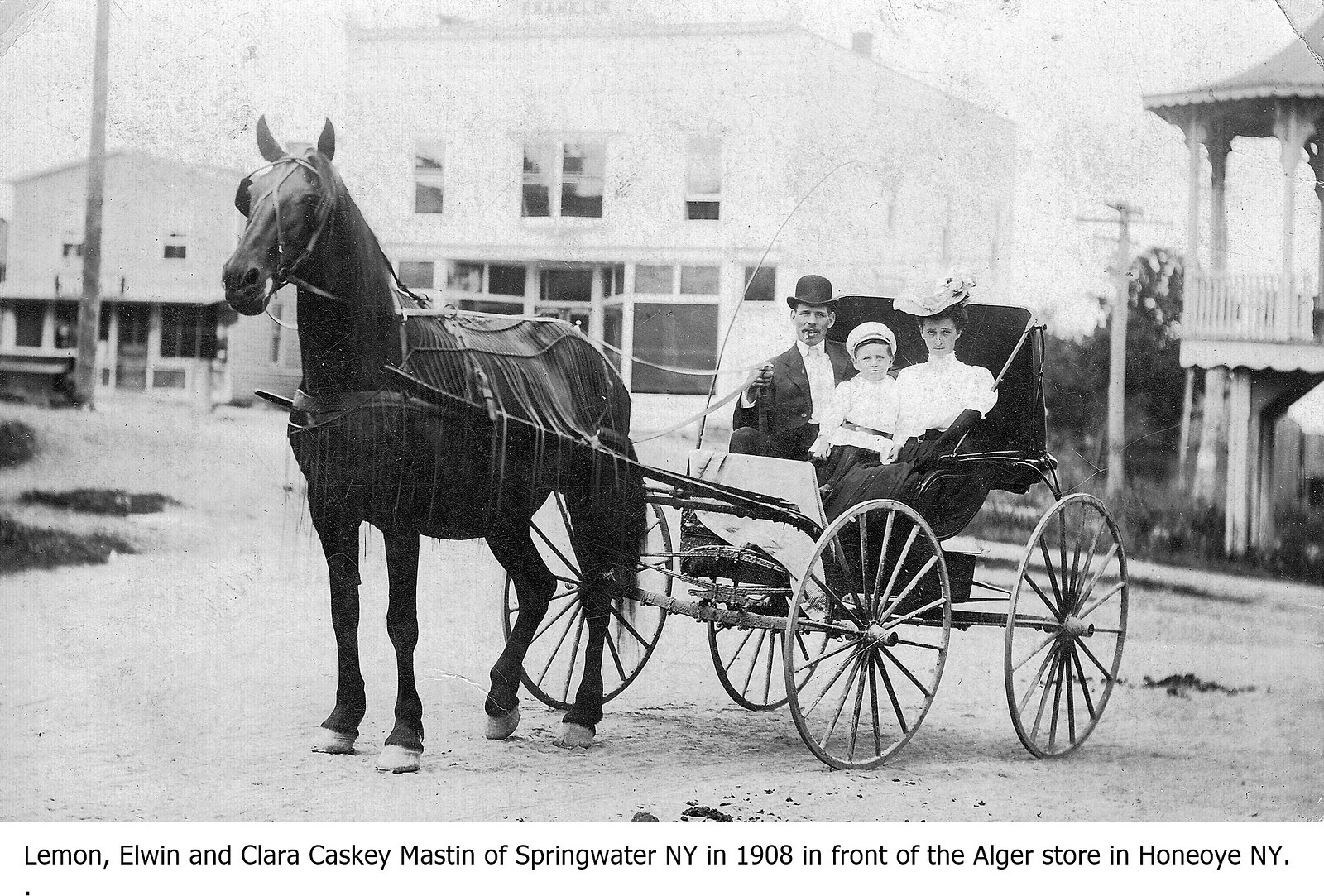The black and white photograph, taken in 1908 in front of the Alger store in Honeyoey, New York, captures Lemon, Elwin, and Clara Kasky Mastin of Springwater, New York. The image centers on a black horse-drawn carriage with four large wooden-spoked wheels. Seated from left to right are a man in a suit, tie, and top hat with a mustache, a young boy in a naval-themed outfit with a white top, and a woman in Victorian attire, donning a large hat with a floral pattern, a white blouse, and a black skirt. The horse, standing upright, has dark fur and is equipped with a brown leather harness and poles attached to its sides. The background features commercial buildings, power lines, and a dirt road, indicating it is daylight.